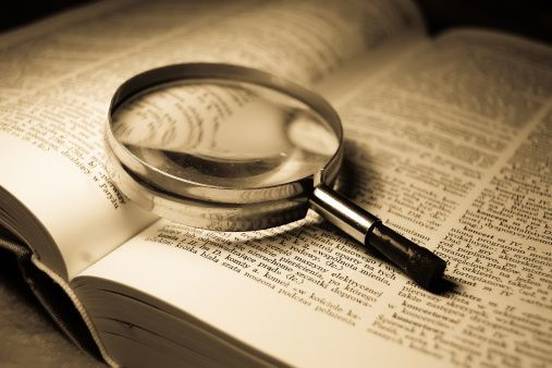In this photograph, a large, open book, which appears to be an index or dictionary, is laid flat against a dark background, with a gradient shading from black at the top to gray at the bottom. The book, seemingly gray-covered, is open about one-fifth of the way through, revealing two white pages filled with two columns of black print, punctuated by bolded words suggesting headers or entries. Spanning across the pages is a large magnifying glass with a silver rim and handle, transitioning to black plastic towards the end. The magnifying glass is positioned within the crease of the book, but despite its placement, the words beneath the glass remain illegible and distorted, hinting at either a possible non-English script or simply the nature of the zoom effect. The entire scene gives a meticulous, scholarly feel through its detailed composition and the subtle play of light and shadow on the magnifier and pages.